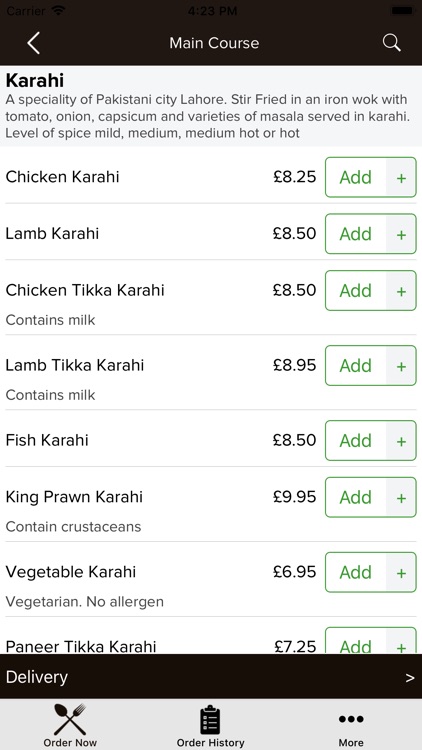This image is a screenshot taken from a mobile phone, showcasing a menu interface. At the top of the screen, there is a large black rectangle with a left-pointing arrow on the left side, labeled "Main Course," and a magnifying glass icon on the right side, indicating a search function. Below this black bar, the background shifts to a clean white.

Centered on the screen, the text "Karahi" is prominently displayed, describing it as a specialty from Lahore, Pakistan. The description highlights that it is a dish stir-fried in an iron wok with tomato, onion, capsicum, and various spices (masala), served with different levels of spice: mild, medium, medium-hot, or hot.

The menu then lists various types of Karahi dishes:
1. Chicken Karahi
2. Lamb Karahi
3. Chicken Tikka Karahi
4. Lamb Tikka Karahi
5. Fish Karahi
6. King Prawn Karahi (noting that it contains crustaceans)
7. Vegetable Karahi
8. Paneer Tikka Karahi

Prices for these dishes are displayed along the right side, appearing in British pounds (£). Each dish listing features a green "Add" button, likely for adding the item to an order.